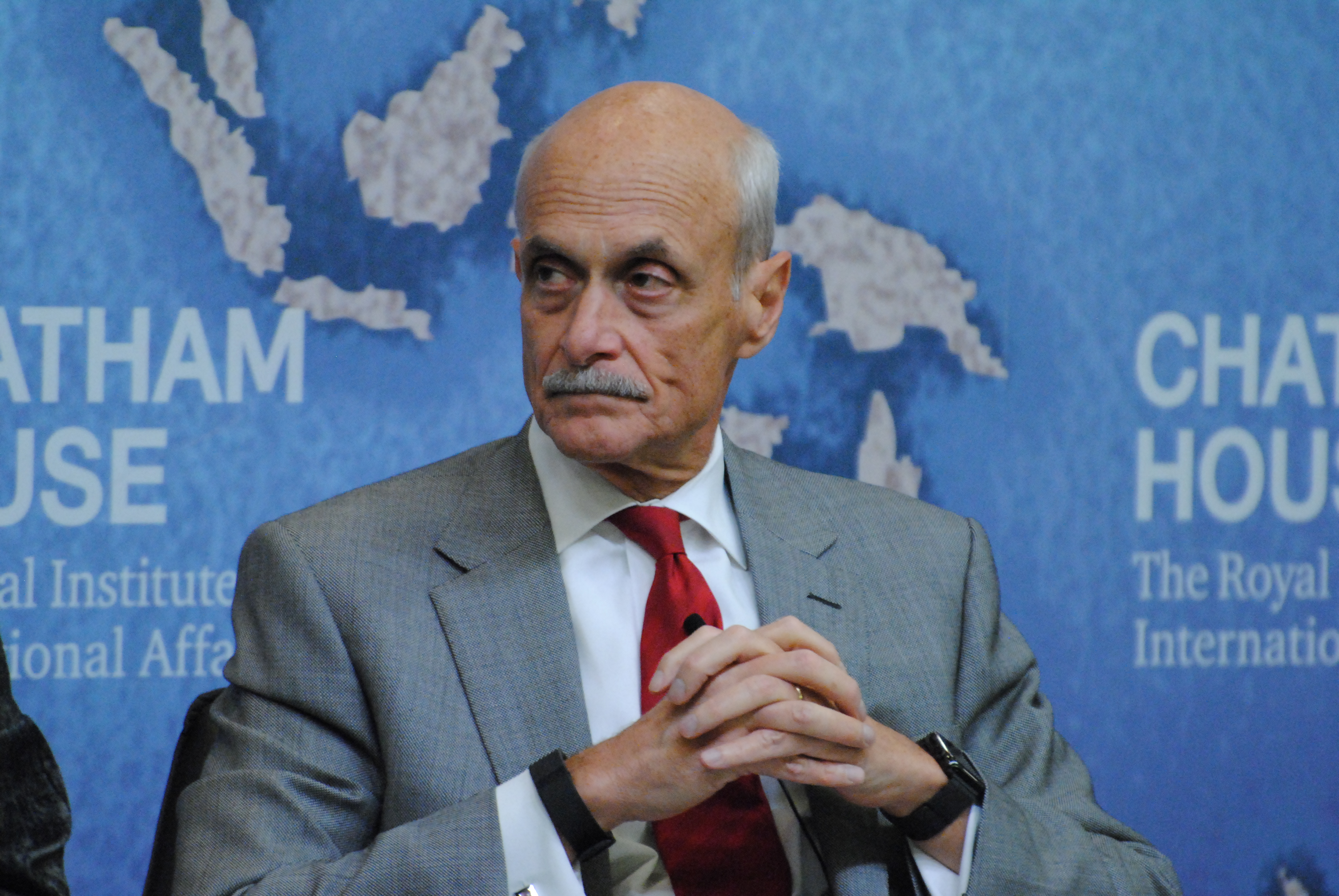This detailed image depicts an older man, likely between the ages of 70 and 75, seated in front of a large, blue map-filled backdrop. He is dressed impeccably in a light gray suit, a crisp white shirt, and a rich red tie tied in a Windsor knot. The man is bald on the top but has gray hair on the sides and sports a matching gray mustache. His demeanor is serious, with his head turned slightly to his right, revealing one pointy ear. He has his hands clasped together with fingers interlaced, resting in front of him, and he wears a watch on one wrist. Behind him, the blue map covers the entire wall, featuring various shades of blue, as well as colors like beige, brown, black, white, and gray. The map includes some partially obscured white text, reading "Chatham House, the Royal Institute of International Affairs," and other cut-off words such as "ATHAM," "USE Institute," and "ENL Affairs."